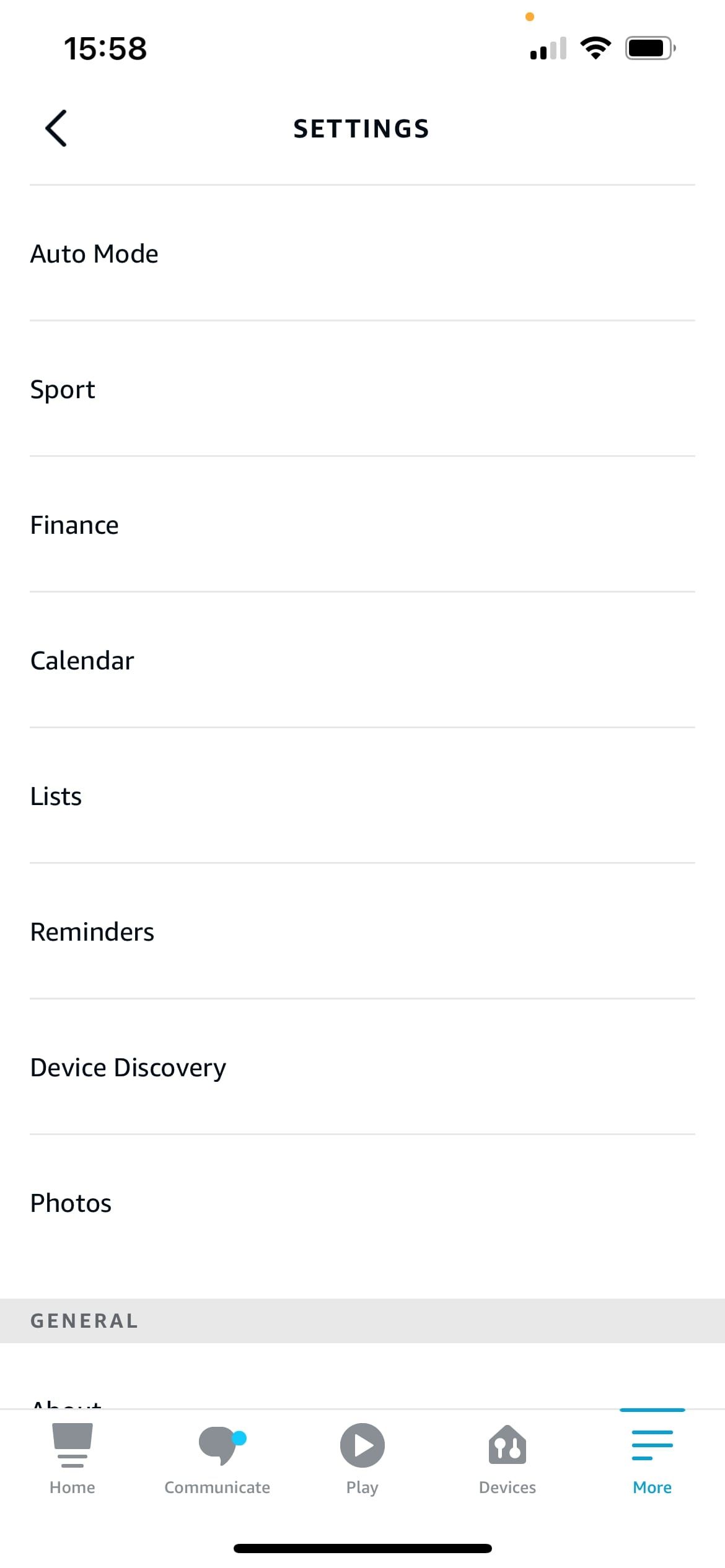The image is a screenshot taken from a phone's settings menu. The screen has a white background, and at the top, the time is displayed as 15:58 in black text. Next to the time are three icons: a cell phone signal indicator, a WiFi signal icon, and a battery symbol displaying a black bar without any numerical percentage.

Below the status bar, the word "Settings" is prominently displayed in black, with a left-pointing arrow icon to its left. The main content area is divided into sections with various settings options listed in a vertical manner.

The initial section includes options such as:
- Auto Mode
- Sport
- Finance
- Calendar
- List
- Reminders
- Device Discovery
- Photos

These options are separated by a light gray divider with the word "General" labeled on the left. Beneath this divider, another line further separates additional settings.

The next section includes:
- Home (accompanied by a distinct symbol)
- Communication (with a small blue or gray dot next to it)
- Play (with a play symbol in the middle)
- Devices (represented by a home symbol)
- More (displayed in blue text)

There are a few lines above these settings, and at the bottom of the screen, there is a thin black bar.

This screenshot captures a comprehensive view of the phone's settings, detailing the various available options and the organizational layout.